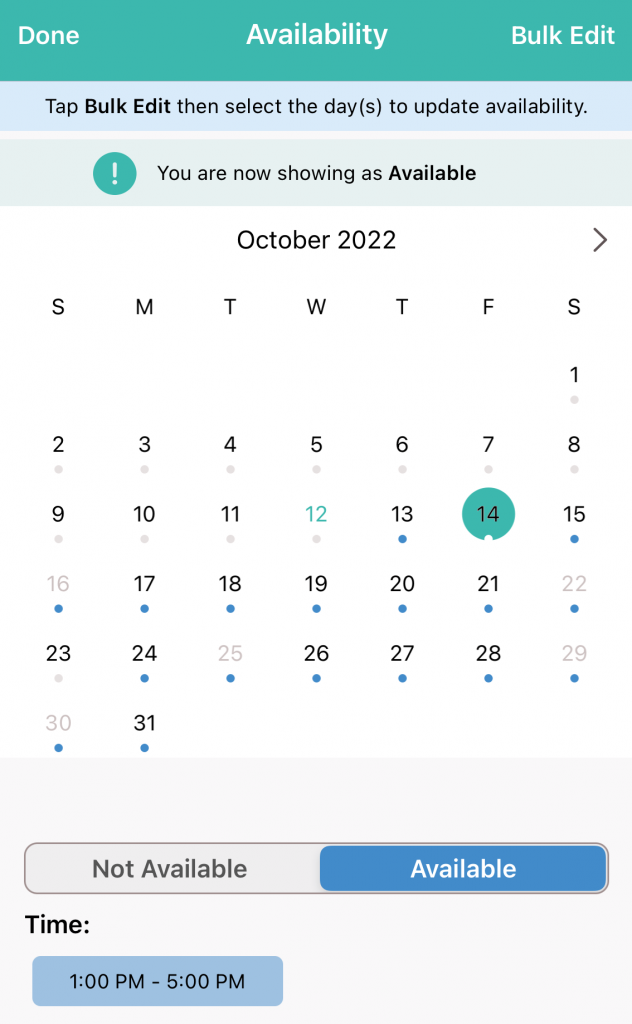This image displays a calendar layout with distinct color-coded sections. The topmost part features a green band, labeled with "Done" on the left, "Availability" in the middle, and "Bulk Edit" on the right. Below this, a blue band advises users to "Tap Bulk Edit and select the day(s) to update availability." Further down, a lighter green section is present.